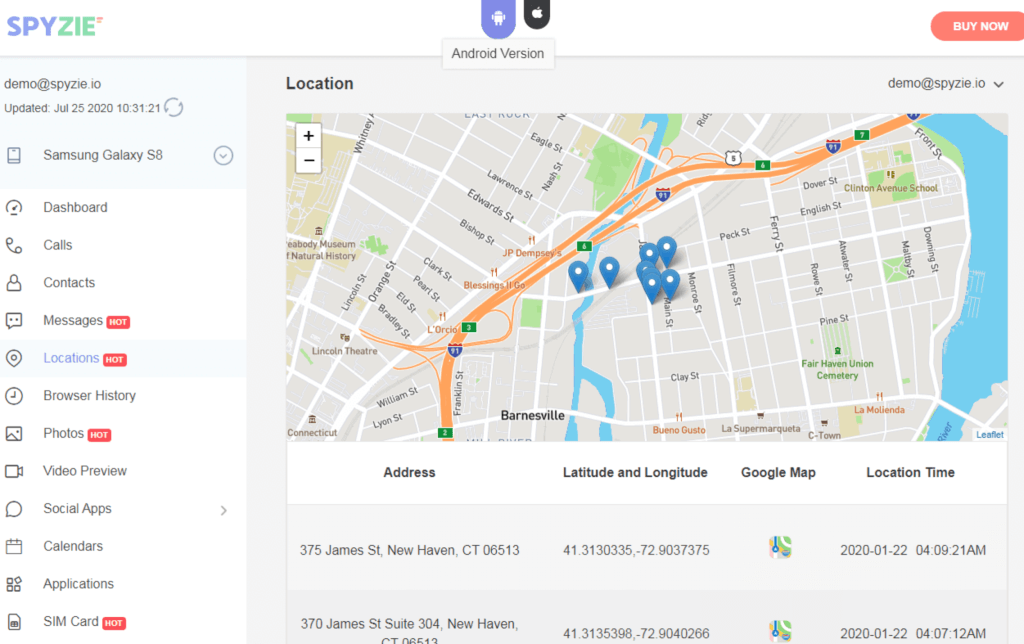This detailed caption describes a screenshot of the Spysy app page:

The screenshot showcases the interface of the Spysy app. In the upper left corner, the Spysy logo is prominently displayed. Below the logo, a left sidebar features a demonstration link titled "demo at spysy.io" and lists a monitored device, "Samsung Galaxy S8," accompanied by a phone icon. The sidebar presents various options, including:

- Dashboard
- Calls
- Contacts
- Messages
- Locations (highlighted)
- Browser History
- Photos
- Video Preview
- Social Apps
- Calendars
- Applications
- SIM Card

Taking up the majority of the right side of the screen is a large, detailed map with the heading "Location" above it. The map features labeled streets such as Eagle Street, Clay Street, and Pine Street. Points of interest marked on the map include "Bueno Gusto" (depicted with a knife and fork icon, indicating it's a restaurant), "La Molienda" (another restaurant), and "Fairhaven Union Cemetery." In larger print at the bottom of the map, the town name "Barnesville" is indicated. Seven blue pins mark various locations across the map.

Below the map, four columns are presented, labelled Address, Latitude and Longitude, Google Map, and Location Time. The first listed address is "375 James Street, New Haven, Connecticut, 06513," followed by its latitude and longitude coordinates, a thumbnail image of the corresponding Google Map location, and the timestamp "2020-01-22 04:09:21 AM." Subsequent rows contain additional addresses with corresponding details.

This comprehensive view provides insights into the array of monitoring features offered by the Spysy app, showcasing both location tracking and detailed logs of the monitored device's movements.